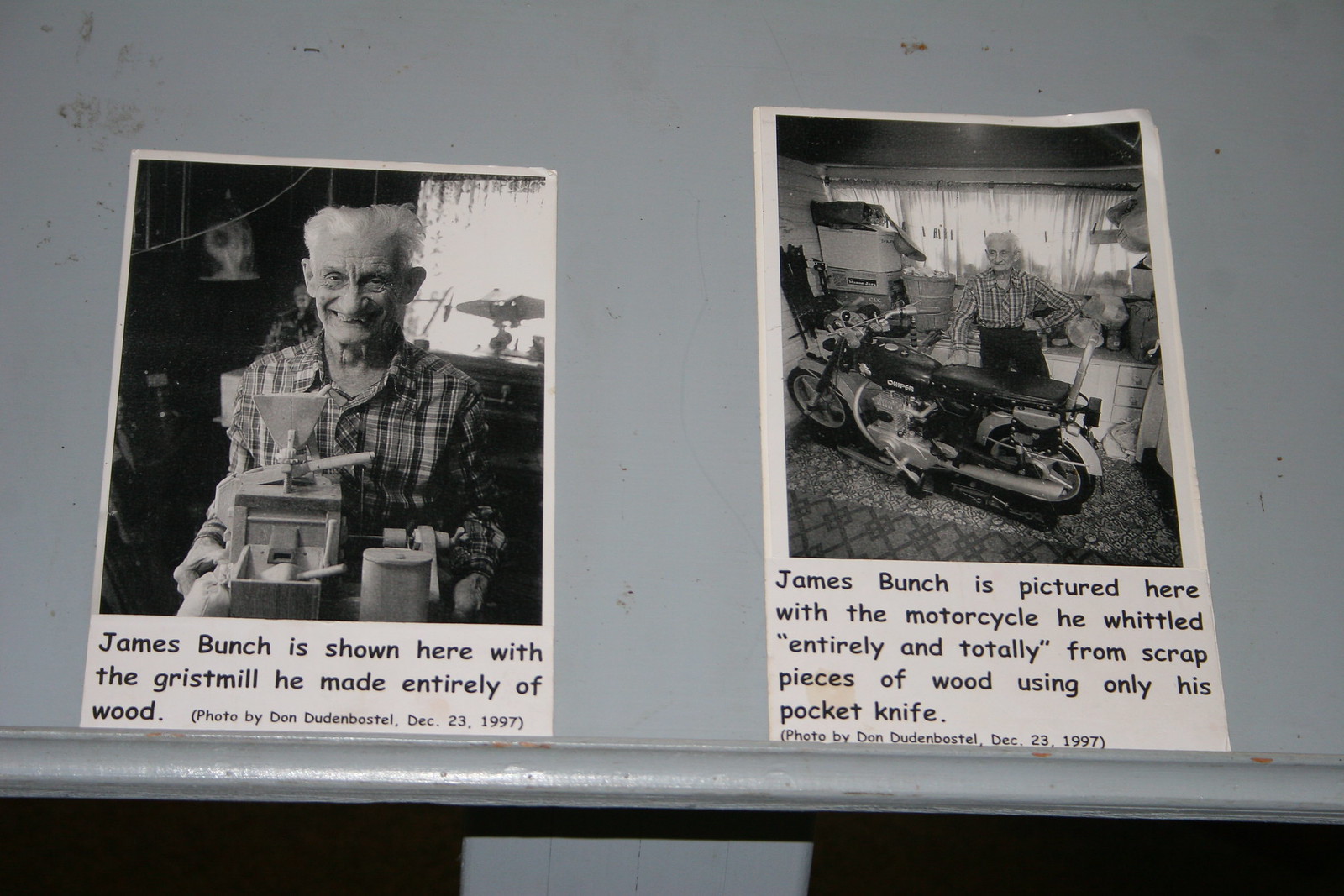This image features two black-and-white photographs mounted against a gray wall, showcasing the craftsmanship of an elderly man named James Bunch. In the left photograph, James Bunch, donned in a plaid shirt, sits proudly in front of a meticulously handcrafted wooden gristmill. The accompanying caption reads, "James Bunch is shown here with the gristmill he made entirely of wood. Photo by Don Dudenbostel, December 23, 1997." On the right, a slightly larger photograph depicts James Bunch standing in his kitchen next to a wooden motorcycle. The second caption states, "James Bunch is pictured here with the motorcycle he whittled entirely and totally from scrap pieces of wood using only his pocket knife. Photo by Don Dudenbostel, December 23, 1997." Both photos capture the pride and skill of James Bunch, underscored by his consistent attire and serene smile.